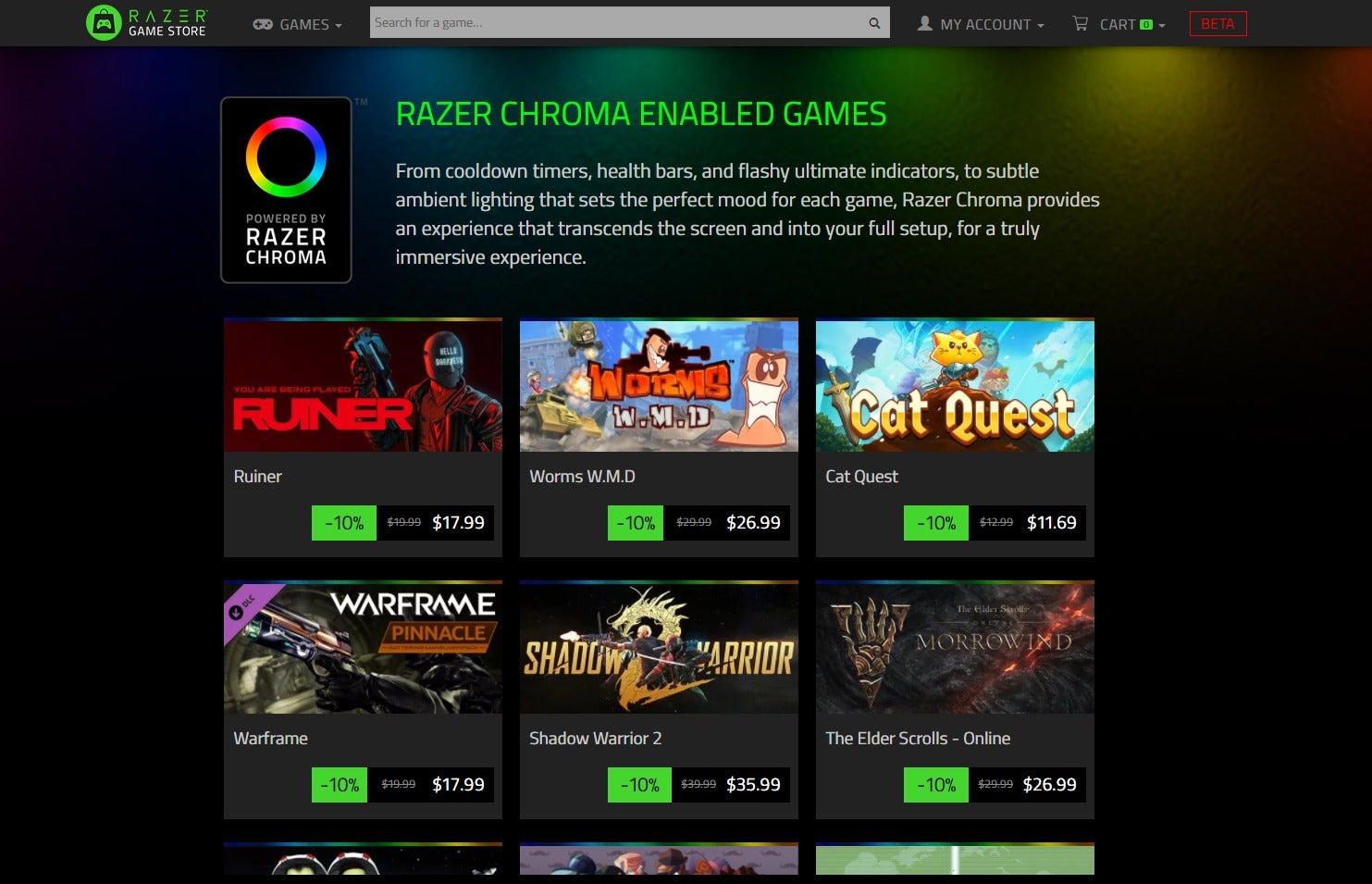The image appears to be a screenshot captured from a computer, showcasing a black background with interface elements. In the top left corner, there's a green circle containing a black square, next to text that reads "Razor Game Store." Immediately to the right, there is a gray square serving as a search bar. Further to the right, the interface features options labeled "My Account" and "Cart."

Dominating the middle section, a bold green title states "Razor Chroma-enabled games." Below, a descriptive paragraph elaborates: "From cooldown timers, health bars, and flashy ultimate indicators to subtle ambient lighting that sets the perfect mood for each game. Razor Chroma provides an experience that transcends the screen and into your full setup for a truly immersive experience."

Beneath this text, are six featured games in two rows. The top row includes:

1. "Runner," discounted by 10%, priced at $17.99.
2. "Worms W.M.D," also discounted by 10%, available for $26.99.
3. "Cat Quest," similarly discounted by 10%, coming to $11.69.

The bottom row features:

1. "Warframe," with a 10% discount, priced at $17.99.
2. "Shadow Warrior 2," discounted by 10%, available for $35.99.
3. "The Elder Scrolls Online," also discounted by 10%, priced at $26.99.

Each game showcases its title, discount rate, and new price, indicating a promotional offer for Razer Chroma-enabled games.